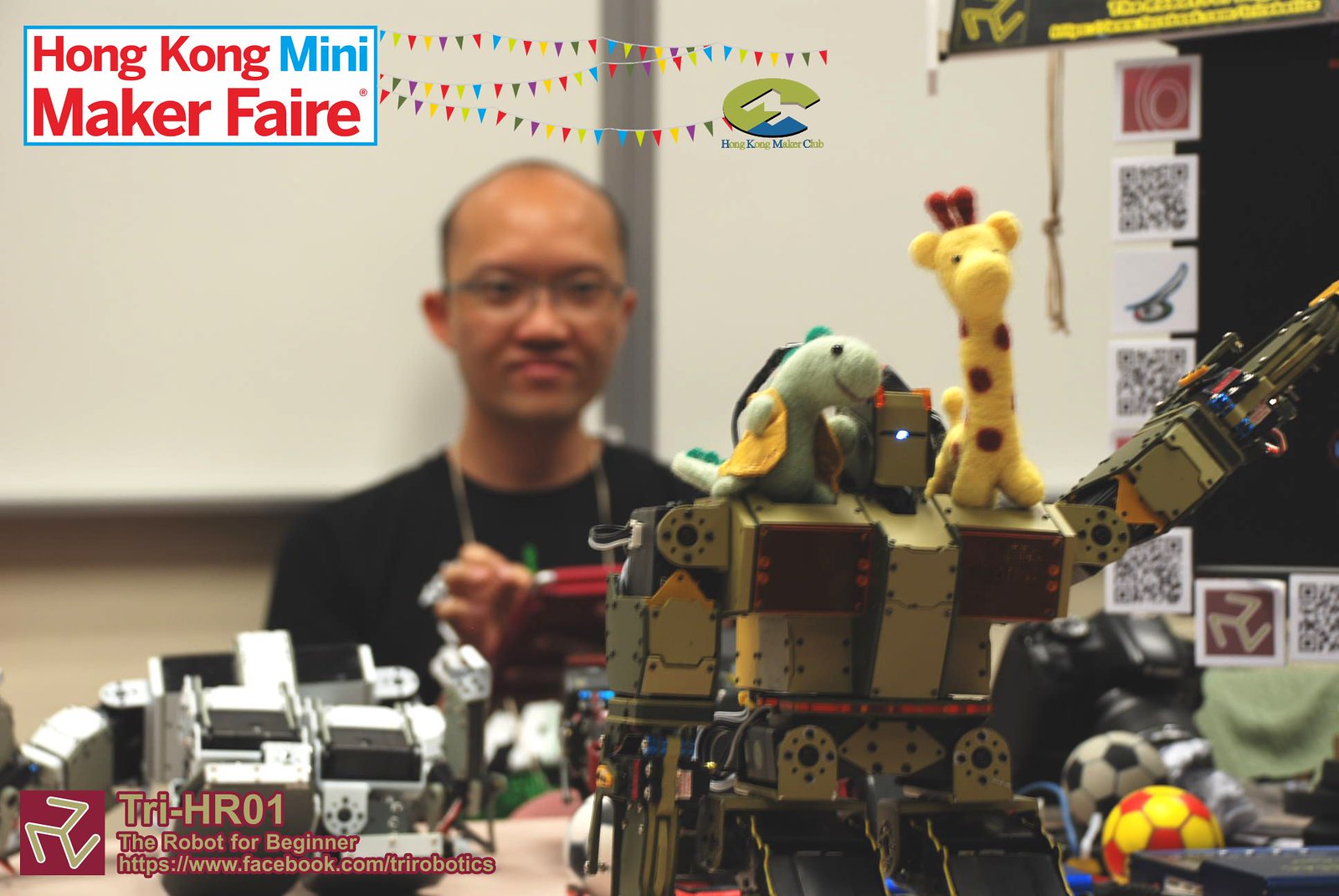The image showcases a promotional scene from the Hong Kong Mini Maker Faire. Dominating the foreground, a variety of toys are displayed, including a plush giraffe and dinosaur, two mini soccer balls—one black and white and the other yellow and red—and several other robotic components. These items are arranged on a robot with an arm extending outward. An Asian male who is balding and wearing glasses is seen in the background, slightly blurry, holding a red remote control, likely to operate the robot for demonstration purposes. The setting is adorned with colorful banners and flags, contributing to the fair's vibrant atmosphere. In the top left corner, a small banner reads "Hong Kong Mini Maker Faire" in multicolored text with a blue-bordered white background. At the bottom left, text and a logo state "Try-HR01, the robot for beginner," alongside a Facebook link to the Tri Robotics page.